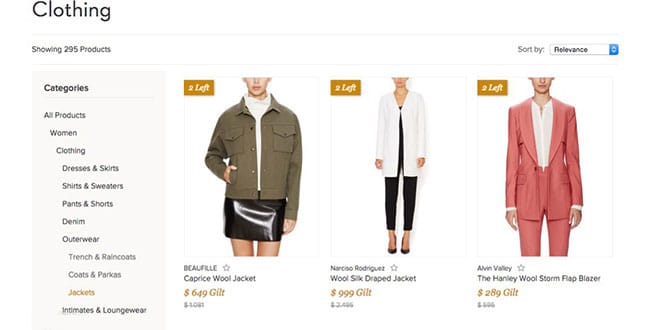**Detailed Caption:**

The image features a variety of women's clothing items categorized into different groups, such as dresses, sports attire, pants, dresses, outerwear, coats, and jackets. This collection appears to be associated with an entrepreneur from Atlanta and includes items like:

- A brown wool jacket from Caprice.
- A white wool silk draped jacket with a unique number, 999, potentially from the brand Nurbidee's Rag-a-noo.
- A pink suit comprising pink pants and a matching pink belt, likely suitable for professional or semi-formal occasions.
- Black pants for a versatile, classic look.
- A black shiny leather skirt for those who prefer a chic and edgy style.
- Multiple white undershirts, ideal for layering or wearing as simple standalone pieces.
- A black undershirt to match various outfits.
- Additional accessories and garments like a wool stove flap, possibly from brands like Gilf, Allerby, or the Herbany.

Among these items are coats and jackets available in shades of brown, white, and pink, indicating a diverse color palette. The text also makes mention of sorting items by preference and suggests saving on selected pieces, emphasizing a tailored shopping experience.

The image prominently displays these garments, focusing on the details such as the mouth, neck, feet, and thighs, providing a comprehensive view of how these clothes fit and appear when worn. The number references such as 999 and 'number left,' suggest inventory details or limited edition items, enhancing the exclusivity of the collection.